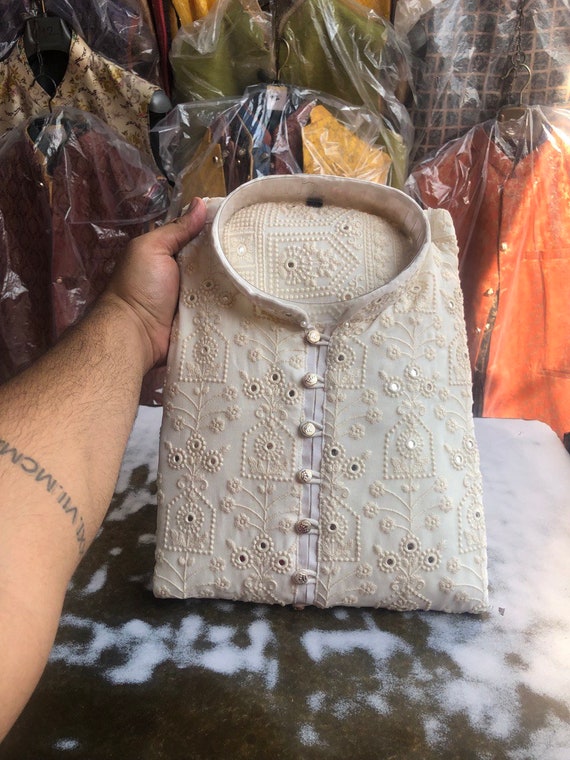The photograph captures a detailed scene involving a cream-colored, ornately embroidered shirt held up by a man's left arm. The man appears to have a medium skin tone with visible dark brown hair and a tattoo in Roman numerals (XXI.VI.MCM). The shirt is meticulously folded, featuring pearl buttons fastened with loops and a stand-up collar reminiscent of a clerical style. The intricate beadwork forms patterns of flowers and geometric shapes, adding to its decorative appeal. The image suggests a retail environment; in the background, various colorful garments—orange, yellow, green, and burgundy—are hung on hangers and wrapped in plastic, possibly to protect them. The shirt is displayed over a worn, brown work table that has patches of white paint and a cowhide-patterned cloth, adding a rustic element to the scene.